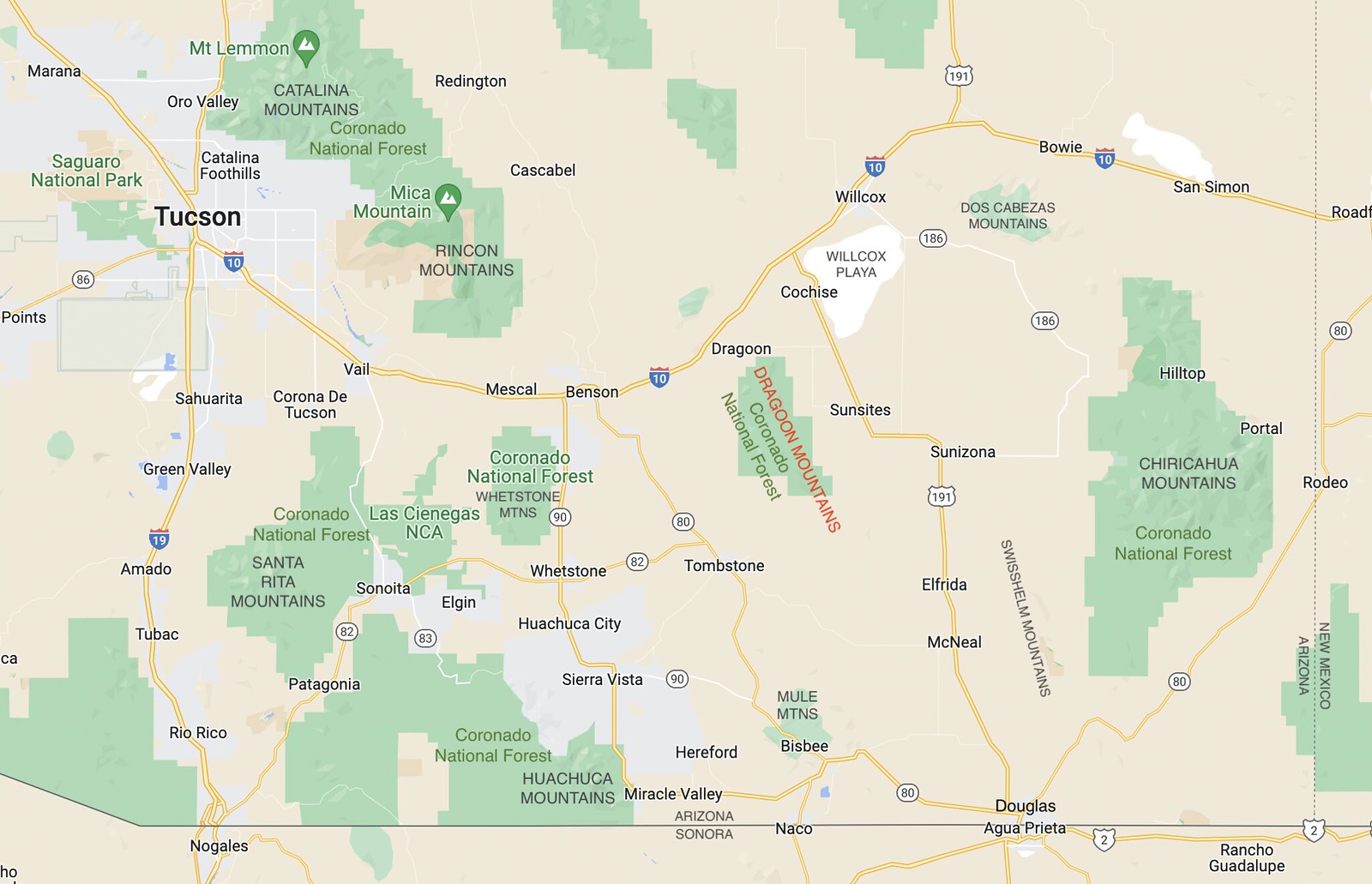The image depicts a detailed, horizontally-oriented rectangular map with a pale pinkish-gray background, predominantly leaning towards a pink hue. The map highlights various geographic features with pale green regions representing forests or mountainous areas. There are no water bodies visible in the image.

Starting from the upper left, the map outlines the Catalina Mountains, part of the Coronado National Forest, including notable landmarks such as Micah Mountain and the Rincon Mountains. This section is one of the larger green areas on the map. Additional green areas are scattered along the top edge of the map.

At the bottom left, the map shows a smaller section of forests and mountains, also part of the Coronado National Forest. Here, the Santa Rita Mountains and La Cienegas National Conservation Area are highlighted. Further to the right, the Whetstone Mountains are identified within another slightly separated part of the Coronado National Forest. Below that, yet another detached section of the Coronado National Forest is noted, with the Huachuca Mountains at the southernmost point.

Smack dab in the middle of the map lies the Dragoon Mountains, also within the Coronado National Forest. On the right side of the map, the Chiricahua Mountains are depicted, belonging to the same national forest, representing yet another significant green area. Despite the presence of these forests, the pink sections dominate the map.

The map also features various roadways, with a prominent swooping road at the top, possibly numbered 70. Several vertical roads run downward from this top road, including routes numbered 19, 191, and 90. Additionally, the map indicates several small towns scattered around these roads, providing a detailed overview of the region.